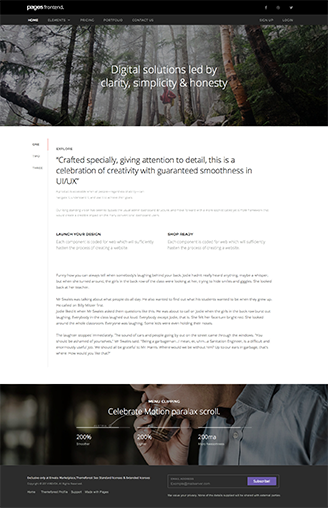Under the category of websites, this webpage features extremely small and difficult-to-read text. At the top, there is a black bar with unreadable text, followed by a smaller bar below it, also containing illegible letters. Due to the tiny font size, enlarging the text is not an option.

Directly beneath these bars is an image depicting a foggy forest scene with trees and shrubbery, along with some rocks on the side. Superimposed on the image in white letters, it reads: "Digital solutions led by clarity, simplicity, and honesty."

Below this text, there is a heading that is indistinct, followed by another phrase stating: "Crafted specially giving attention to detail." It continues with: "This is a celebration of creativity with guaranteed smoothness in UI/UX."

Further down, there are a couple of unreadable paragraphs. At the bottom of the page, it encourages users to "Celebrate motion and parallax scroll." Additionally, there is an image of a man drinking from a very small cup.

This webpage appears to emphasize innovative digital solutions with a focus on simplicity, clarity, and user-friendly design elements, highlighted by an artistic, nature-inspired visual theme.